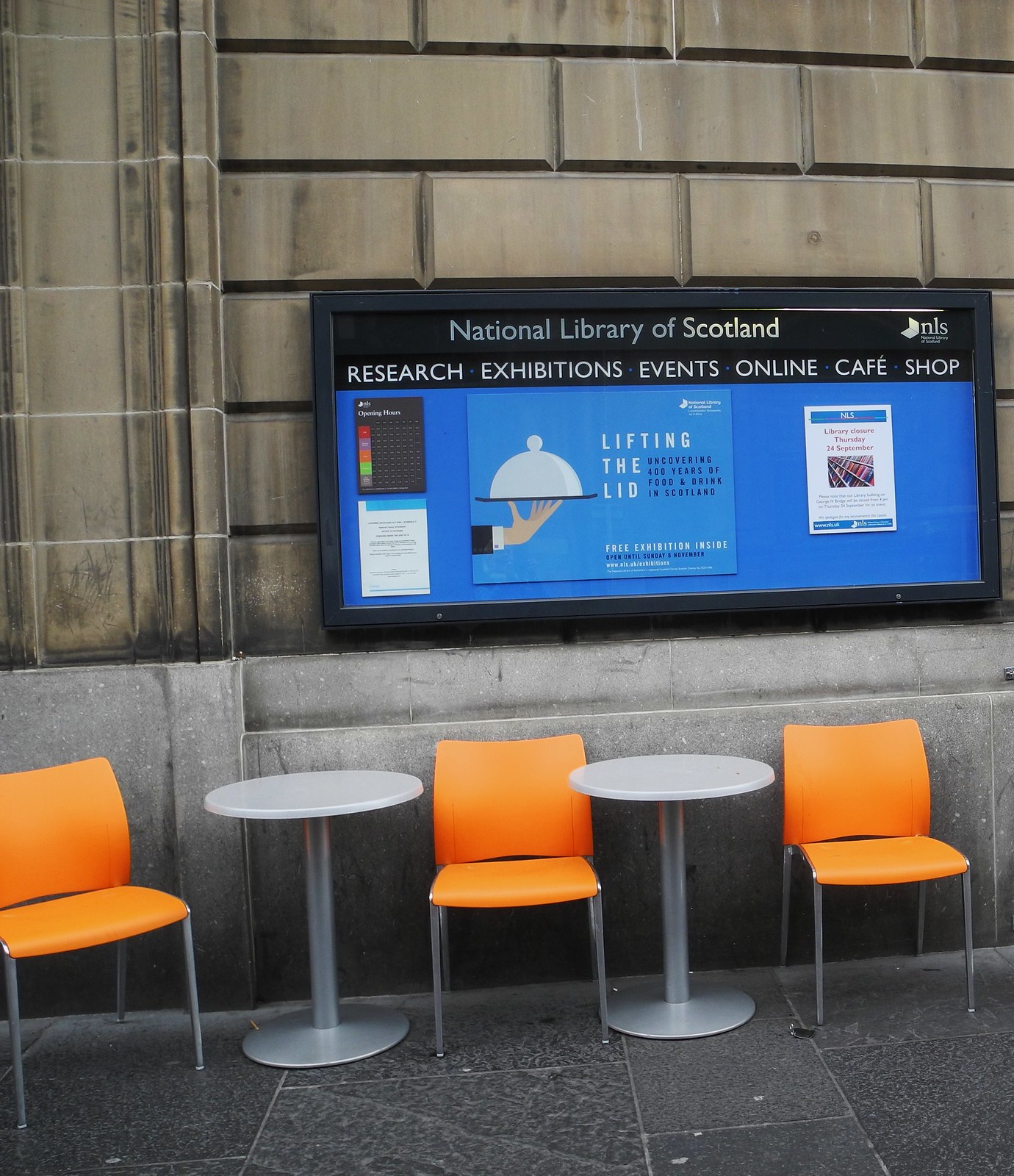The photograph captures the exterior of the National Library of Scotland, showcasing its imposing stone-tiled facade with a concrete base. Prominently displayed on the wall is a large sign that reads "National Library of Scotland" followed by the services offered: Research, Exhibitions, Events, Online, Cafe, and Shop. Beneath this header are three posters. The left poster features a calendar with Opening Hours, and the middle poster, adorned in blue, showcases an event titled "Lifting the Lid: Uncovering 400 Years of Food and Drink in Scotland," with a cartoon hand holding a covered platter. The right-hand poster announces a library closure on Thursday, 24th of September. In front of the sign, there are two small round tables with aluminum pedestals, flanked by three orange plastic chairs, inviting passersby to sit and relax.